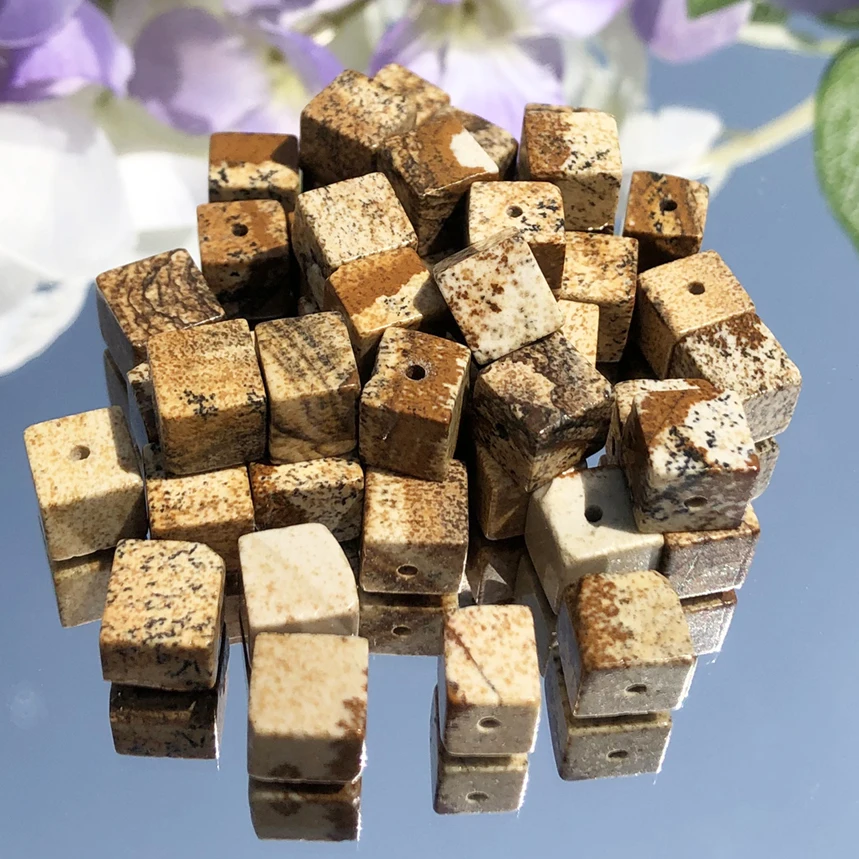The image depicts a collection of small square blocks that appear to be made from a hard material resembling granite or wood. These blocks, each featuring a round hole through the center, are arranged in a complex pattern. The majority are darker brown, with some in lighter shades of cream and beige, all exhibiting speckled or splotched designs akin to granite. They are positioned on top of a glass-like surface, reflecting their forms. The arrangement shows the blocks being stacked, with heights varying from five or six high in the back to two or three high in the front. The backdrop contains blurred light purple flowers and a semicircle of a green transparent object against a solid blue background. Additionally, there seems to be an artistic depiction of a tree in violet and dark purple with streaks of green and white, appearing to float above the blocks.